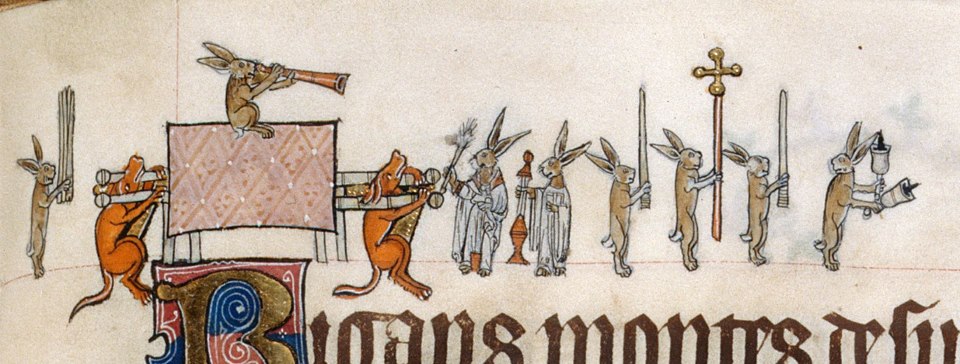This detailed drawing depicts a procession of light brown rabbits engaged in what appears to be a religious or ceremonial ritual. At the forefront, several rabbits stand upright in a row, each holding objects such as sticks, crosses, and incense burners or candles. The lead rabbit is ringing two bells, seemingly to alert others about the ongoing parade. Behind them, two notable rabbits are dressed in ceremonial robes, extending to their feet, with one holding a staff in its right hand. Their ears are prominently upright. On the left side of the image, two dark brown animals, likely foxes or dogs, are shackled to a wheeled carrier, their bodies hanging down. Atop this apparatus, a rabbit blows a horn, possibly signaling the procession's movement. The background of the image is a very light brown, and at the bottom, there is partially visible text written in dark brown calligraphy, further enhancing the mystique of the scene.